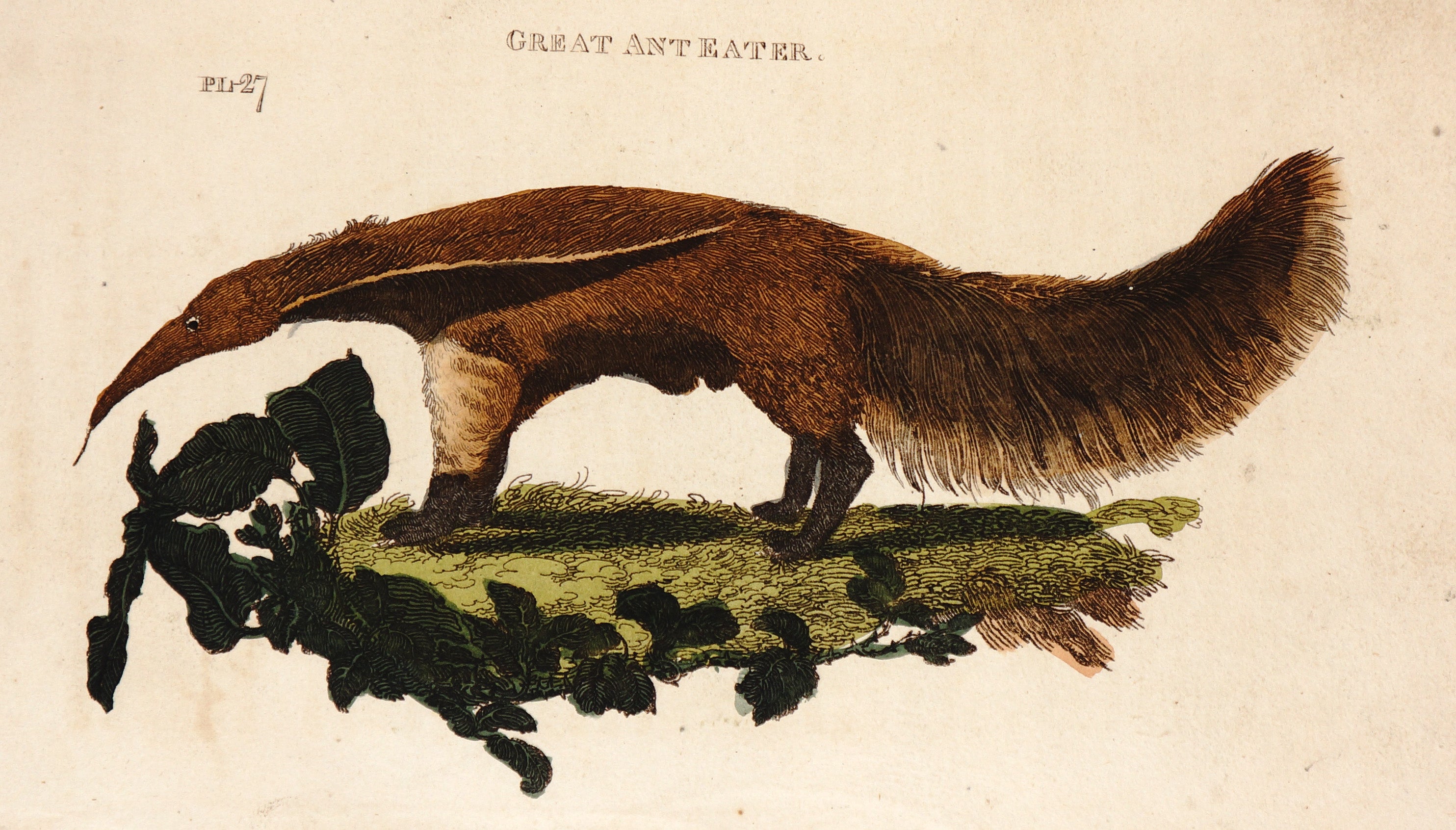This detailed illustrative diagram of the Great Anteater is set against a worn, cream-colored parchment background. The top of the image is labeled "Great Anteater" in brown text, with "PL 27" slightly below and to the left. The anteater is depicted standing on a small grassy area with a few leaves silhouetted in dark tones on the left. The image portrays a detailed side profile of the anteater, which predominantly features a reddish-brown furry body. Noteworthy is the beige color on the top of its front left leg, contrasting with the black coloring on the bottom of its feet and the back legs from the knee down. The anteater's head is turned to the left, displaying its distinctively long, pointed face with a small, string-like tongue extended outward. The eye of the anteater is detailed with a small white area and a large black pupil. Extending from the right, the tail is a dark brown, exceptionally shaggy, and slightly lighter at the ends, curving up and then down to create a flowing, textured appearance.